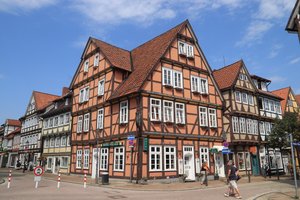In this image, we see a charming intersection dominated by an orange, peach-colored building with distinct German or Scandinavian architectural features, including a pitched roof and brown trimming. The structure has a total of four rows of windows, distributed as follows: one window at the very top, four windows on the second level, five on the third level, and three windows plus a door on the ground level. The building stands prominently at the corner, showcasing two of its sides in a three-dimensional perspective. Situated in the middle of the image, a pedestrian can be seen crossing the street, adding life to the tranquil scene. The streets, which may be pedestrian walkways as suggested by blockades and the absence of vehicles, form a network radiating from the corner. Surrounding this main building are other similarly designed houses with numerous windows. A lone tree stands on the far right side, enhancing the quaint atmosphere. The sky above is a clear blue, adorned with faint white clouds, emphasizing the serene, lovely day captured in the photograph.